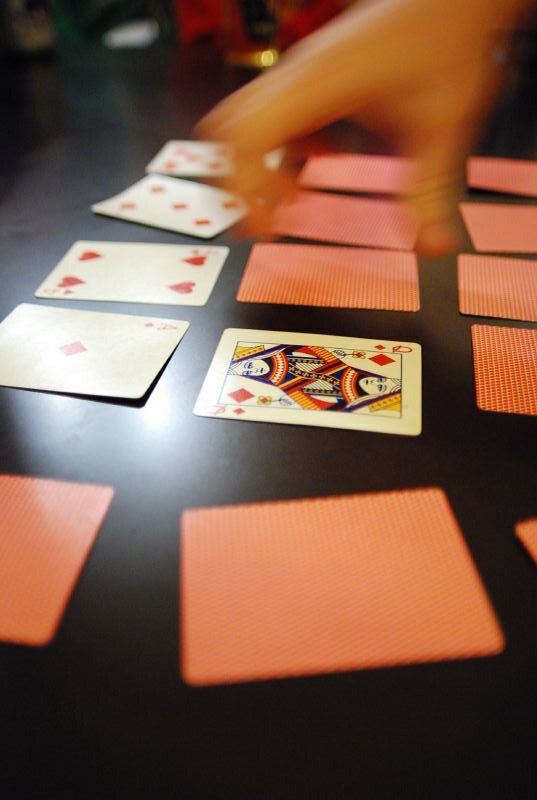This tall photograph prominently captures a scene of playing cards meticulously arranged on a glossy black table, organized in three rows. Each row holds five cards, although only part of the bottom row is visible. The orientation of the cards appears perpendicular to the viewer, meaning the typical top-to-bottom layout of the cards translates into a left-to-right arrangement for the observer.

In the top row, starting from the left, the first card is face down, followed by an Ace of Diamonds, a Four of Hearts, a Five of Diamonds, and finally another Five, the suit of which remains hidden. The middle row also begins with a face-down card, succeeded by a Queen of Diamonds that stands out clearly, with the next three cards all face down. The bottom row, partially obscured, consists only of visible face-down cards, with the corner of an additional card peeking into view on the far right.

Distinctly, a blurred hand appears hovering over the Queen of Diamonds or the card immediately to its right, fingers splayed as if poised to pick up or turn over a card, suggesting an active moment in a game of solitaire.